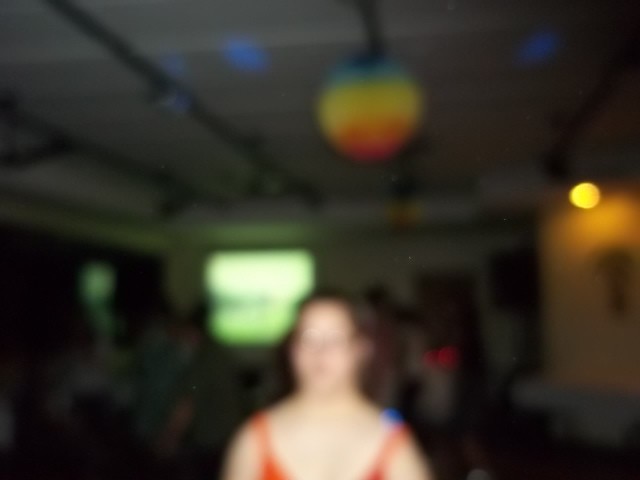The image depicts a dimly lit scene with several distinctive elements. Across the top of the ceiling, there are black vertical lines. Hanging from the ceiling is a circular object featuring multiple colors: red, green, yellow, orange, and red. Additionally, there are a few blue circles adorning the ceiling, which also appears to have some rectangular white pieces scattered across it.

In the background along the back wall, a green element is visible, possibly glowing. To the right of this green section, there is a prominent yellow circle. In the foreground stands a woman, or a person, positioned in front of the green light. She is dressed in a red tank top and has dark hair that is pulled back. The remainder of the background is predominantly dark and out of focus, adding to the overall obscure and blurry nature of the image.